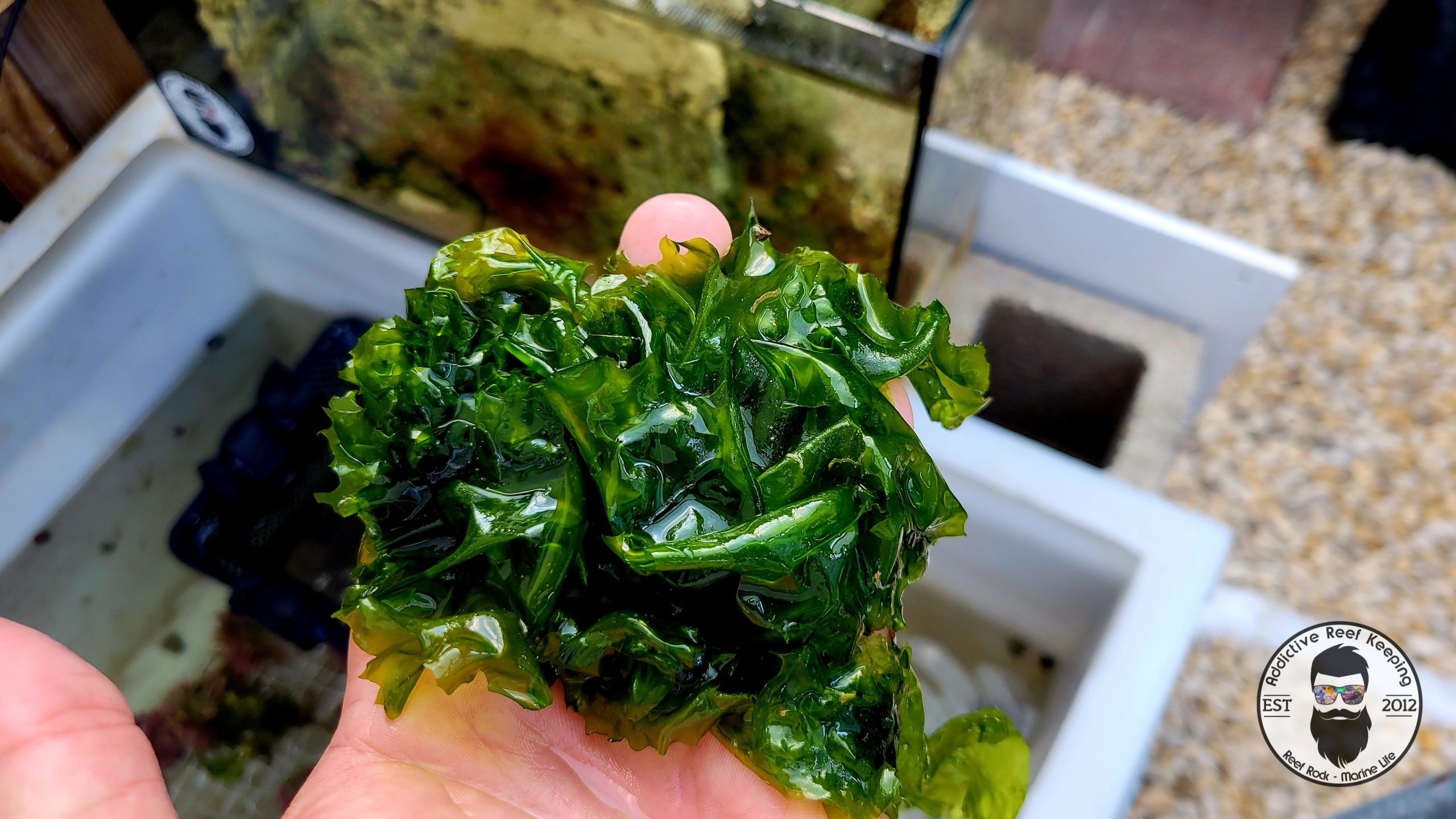This detailed image captures a close-up of a light-skinned person extracting what appears to be vibrant green seaweed or possibly kelp from a water-filled container, somewhat resembling an aquarium. The hand holding the seaweed is prominently featured, highlighting the detailed texture and color of the plant. The surrounding area includes similar containers and stones scattered on the ground, reinforcing the notion of a productive aquatic environment. In the lower right corner, there is a logo featuring an illustrated man with dark hair, a long beard, a mustache, and bombardier-style glasses. The logo, accompanied by the text "Productive Reef Keeping, established 2012," suggests this is part of an established effort in marine cultivation.